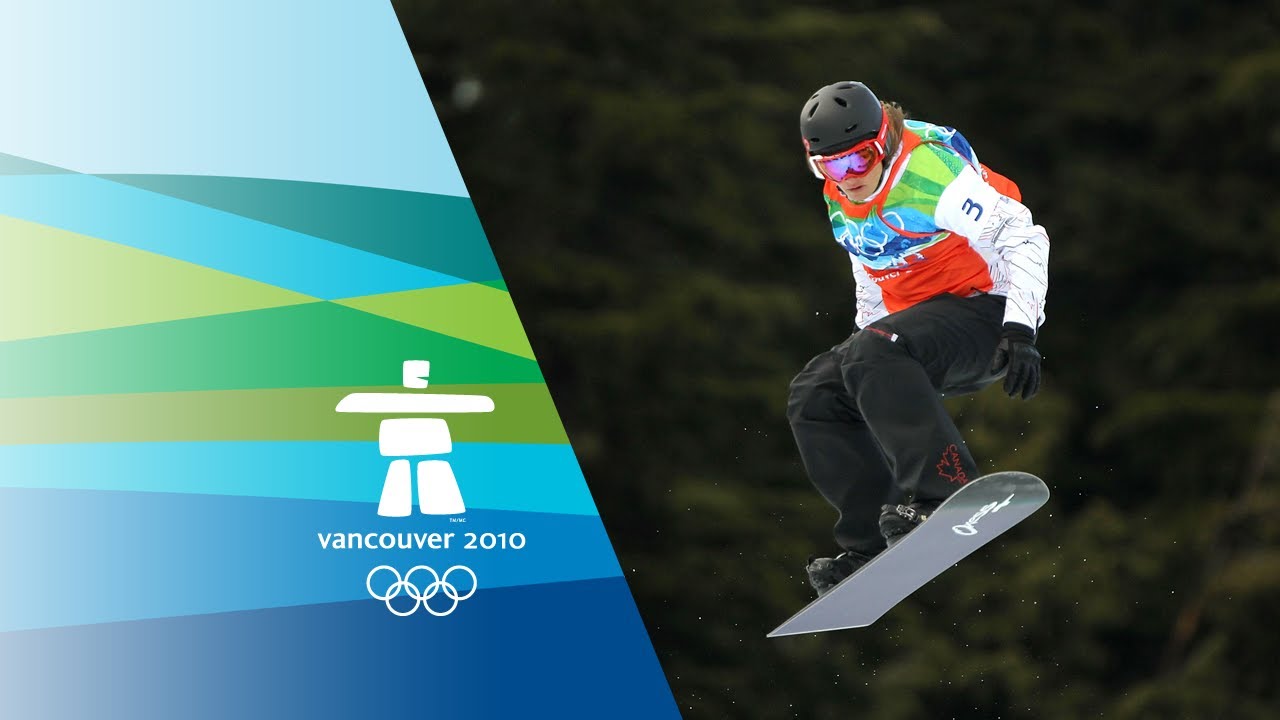The image is divided diagonally into two sections: a digital graphic on the left and a photograph on the right. The left side features a series of geometric shapes predominantly in shades of blue, interspersed with three green shades in the middle. At the top, there's light blue transitioning into aqua green and then light blue again, forming a parallelogram and then a green triangle. The bottom part is dark blue. Over these colors, a white logo of a human figure with arms extended is prominently displayed, beneath which "Vancouver 2010" is written. Below this, the iconic five interlocking Olympic rings can be seen in white. On the right side, a dynamic photograph captures a snowboarder in mid-air, performing a trick. The snowboarder is equipped with a black helmet, red goggles, black pants, and a colorful top featuring a green, red, and blue design. The top also displays an armband with the number three. In the background of the photograph, green trees can be seen, providing a vivid contrast to the action in the foreground.